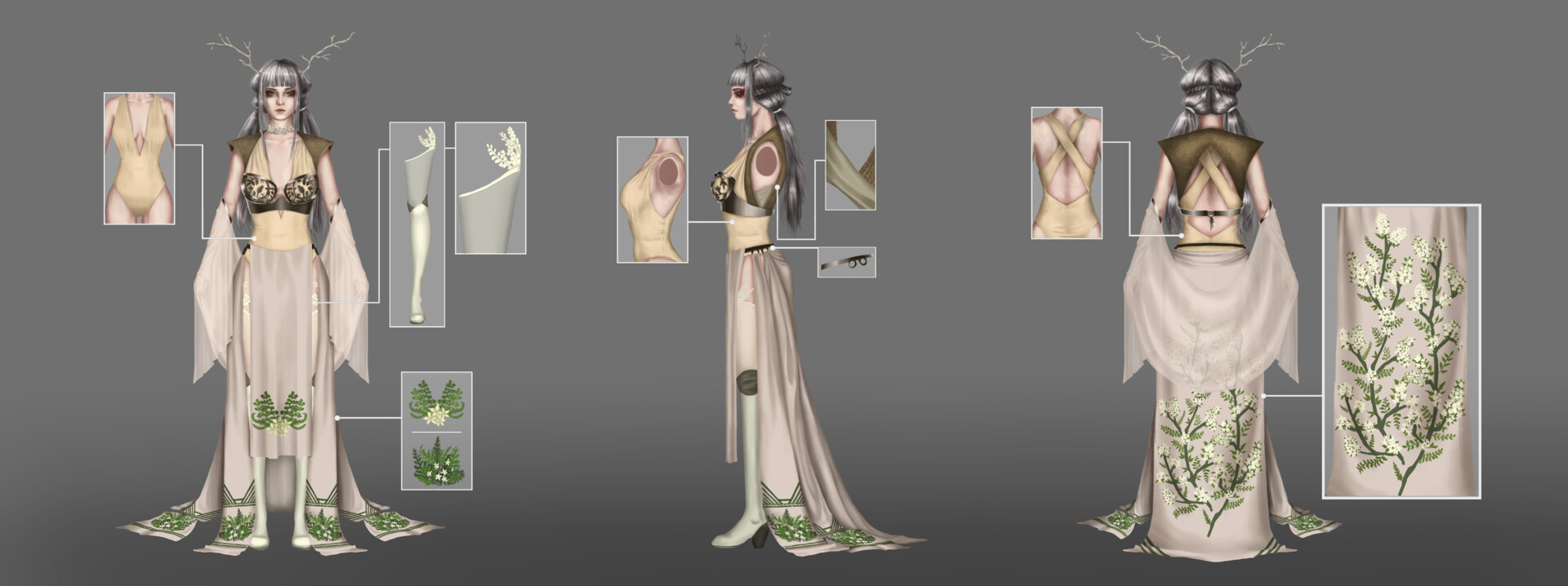This color illustration showcases a detailed 3D render of a woman adorned with intricate, fantasy-inspired attire and headgear resembling deer antlers or branching antlers. The render is composed of three distinct views: front-facing, side-facing left, and back-facing. 

In the front view, the woman has grayish-white, back-length hair and is dressed in a flowing, beige-pink dress with floral embroidery. Her outfit features a unique combination: brown shoulder pads that don’t connect to the main dress, and a gold center section with black breastplates wrapping around her torso. The dress drapes elegantly, revealing greenish-yellow leggings with gray and lighter gray sections, detailed with floral patterns, underneath. Her olive skin provides a contrasting backdrop to her elaborate ensemble.

The side view shows this character turned to her right, highlighting the same costume from a different perspective. A small box illustration reveals an up-close look at the intricate floral embroidery at the bottom of her dress.

The back view illustrates the ornate floral design on the lower part of her dress in greater detail, including white flowers and green stems woven into the fabric. Unique to this perspective, the back straps of her leotard can also be seen, adding to the complexity of her attire. Small supplementary illustrations provide close-ups of the botanical motifs.

Overall, this illustration offers a comprehensive exploration of a fantastical character's costume from multiple angles, emphasizing the sophisticated details and thematic cohesion of her attire.